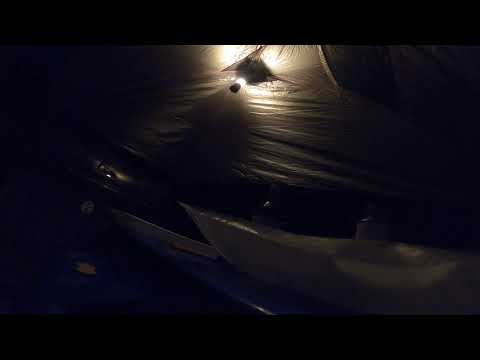In this dark nighttime photograph, there is a square composition dominated by a murky black sky, pierced by a solitary ray of light positioned near the top center. Below, indistinct structures occupy the bottom, exhibiting blurry, ambiguous shapes that evoke the appearance of bananas. These forms hint at blue and white colors but remain difficult to conclusively identify. Some speculate these could be elements within a confined space, possibly inside a tent, shrouded in a thin, dark fabric. The tentative setup suggests a small horizontal scope of around five or six feet, with no discernible presence of people, animals, or vehicles. The enigmatic scene might depict the inside of a tent illuminated by an external light source, or perhaps the side of a boat on a dark lake, accompanied by ripples of water. The primary colors observed include black, brown, white, and a yellowish-white from the distant light, blending into an overall mysterious and indistinct nighttime setting.